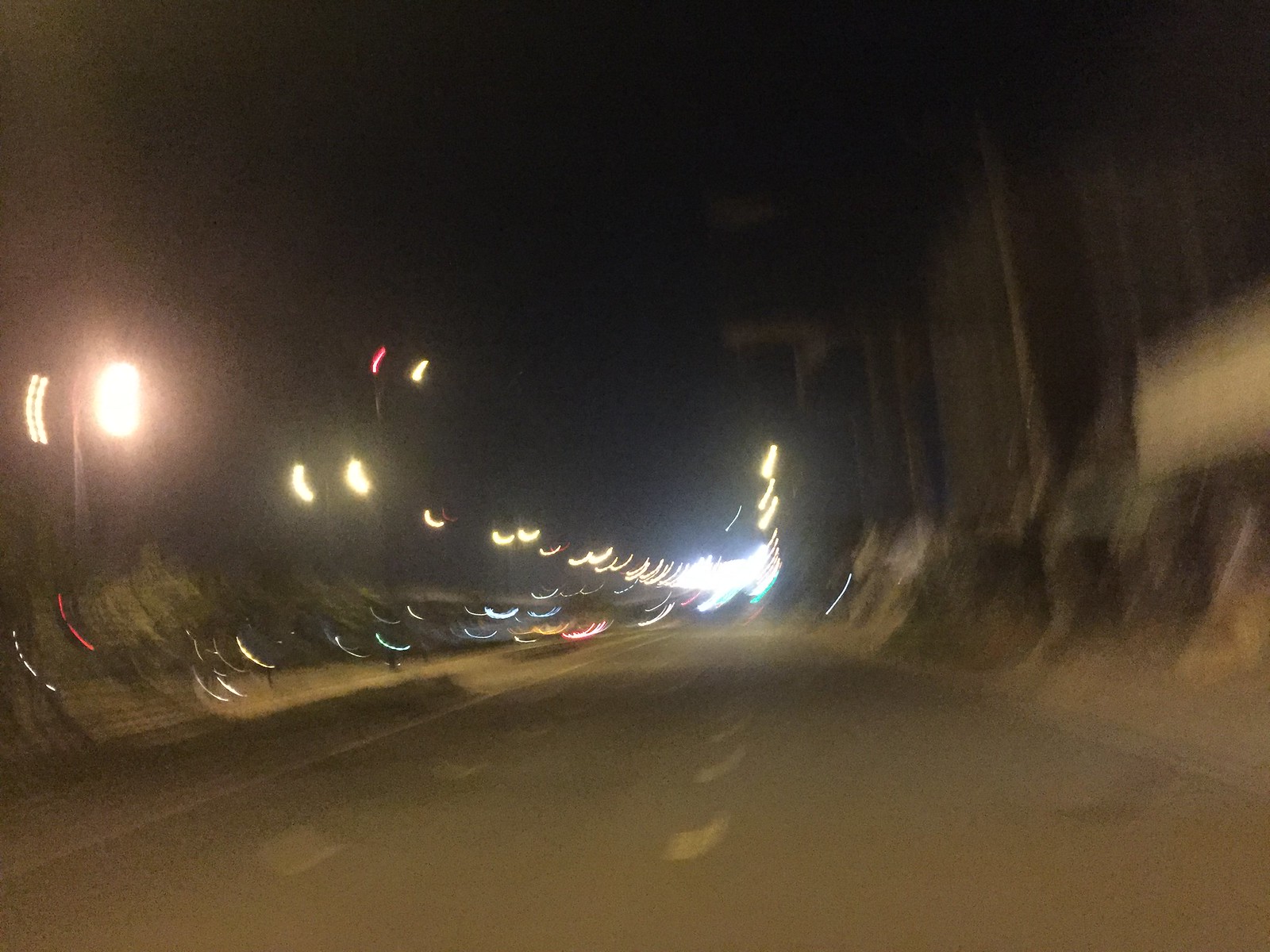This is a very blurry color photograph taken at night, depicting a city street enveloped in strong motion blur. The street, which has two lanes and yellow dashes marking the road, stretches through the center of the image. On the left side, a series of tall street lights, each featuring lights on either side of a vertical pole, create long trails of light due to the motion blur, giving an illusion of numerous lights. The right side of the image suggests the presence of some unlit buildings, and there is a hint of a sidewalk area possibly containing benches. The sky is black, and the overall lack of discernible details results in no visible people, animals, signs, cars, motorized vehicles, plants, flowers, or trees in this photograph.